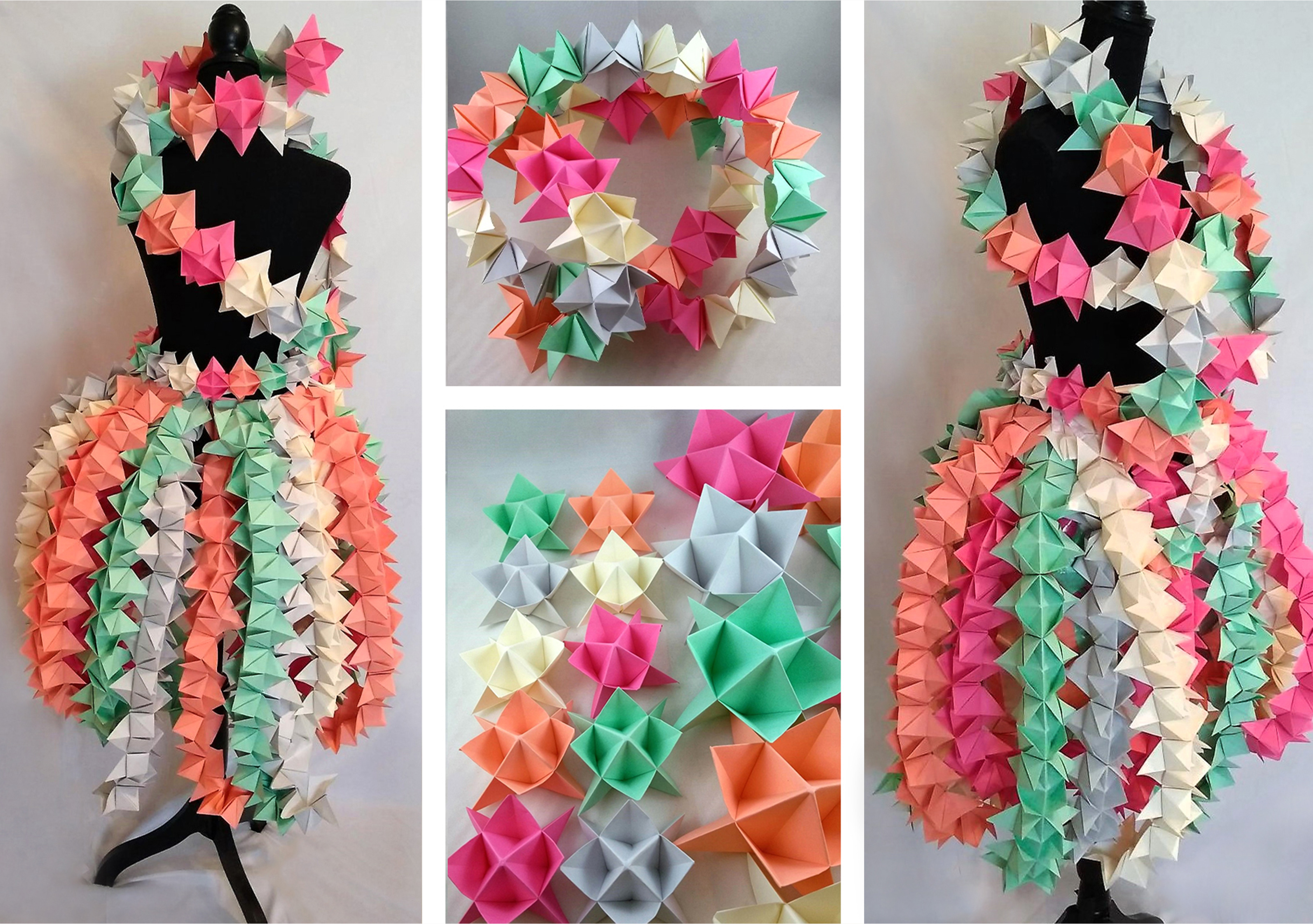The image is a detailed display of origami art fashioned into a dress on a black, headless mannequin. The exhibit is composed of four pictures arranged to highlight different perspectives and close-ups. The two large images on the left and right depict the front and back views of the mannequin adorned with intricate origami pieces forming a skirt, a decorative necklace, and straps crossing the chest and back. These origami pieces resemble interconnected fortune tellers in colors such as pink, orange, pale yellow, light gray, light blue, turquoise, salmon, and white. The middle section includes a close-up of the necklace or lei detail at the top and the individual folded origami components at the bottom, showcasing the craftsmanship before assembly. The display captures the elegance of origami fashion, emphasizing its multifaceted and colorful artistry.